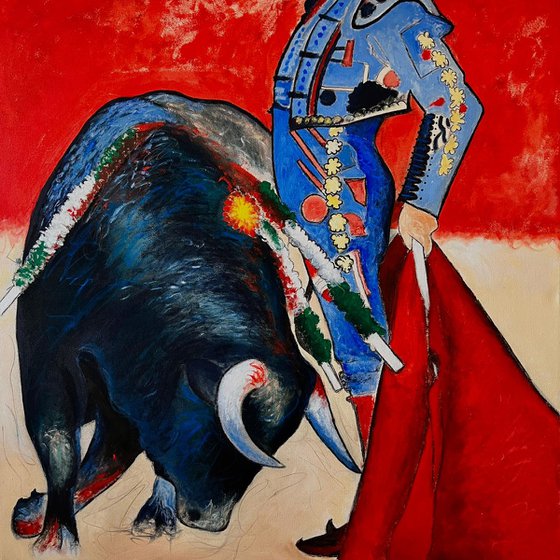The image is a vibrant painting that depicts a dramatic bullfighting scene. The scene is square in orientation and features the matador on the right, whose head is not visible as it is cut off at the top of his shoulders. The matador is facing left, with his front and feet clearly directed to the left. His arms are positioned behind his back, gripping a deep red bullfighting cloth (Olé blanket) that has a white handle. He is dressed in an elaborate sky-blue outfit adorned with both darker and lighter shades of blue along with red stripes and symbols. Notably, yellow stars run along the sides of his waist and down part of his thighs and arms, complemented by floral patterns and red accents on his sleeves. The matador's costume also features epaulets on the shoulders.

To the left of the matador is the bull, which occupies nearly half of the painting. The bull’s shiny black coat reflects various shades of blue and green. The bull's head is down and its curved white horns, stained with blood, are making contact with the matador's lower leg. The bull wears a white strap with green and red sections, which might symbolize additional injuries. The bull's two visible front legs are also marked with red, indicating blood. The background features a striking red wall in the upper third of the image, contrasting with the beige flooring that mimics the arena's sands, creating a vivid and intense depiction of the bullfighting moment.